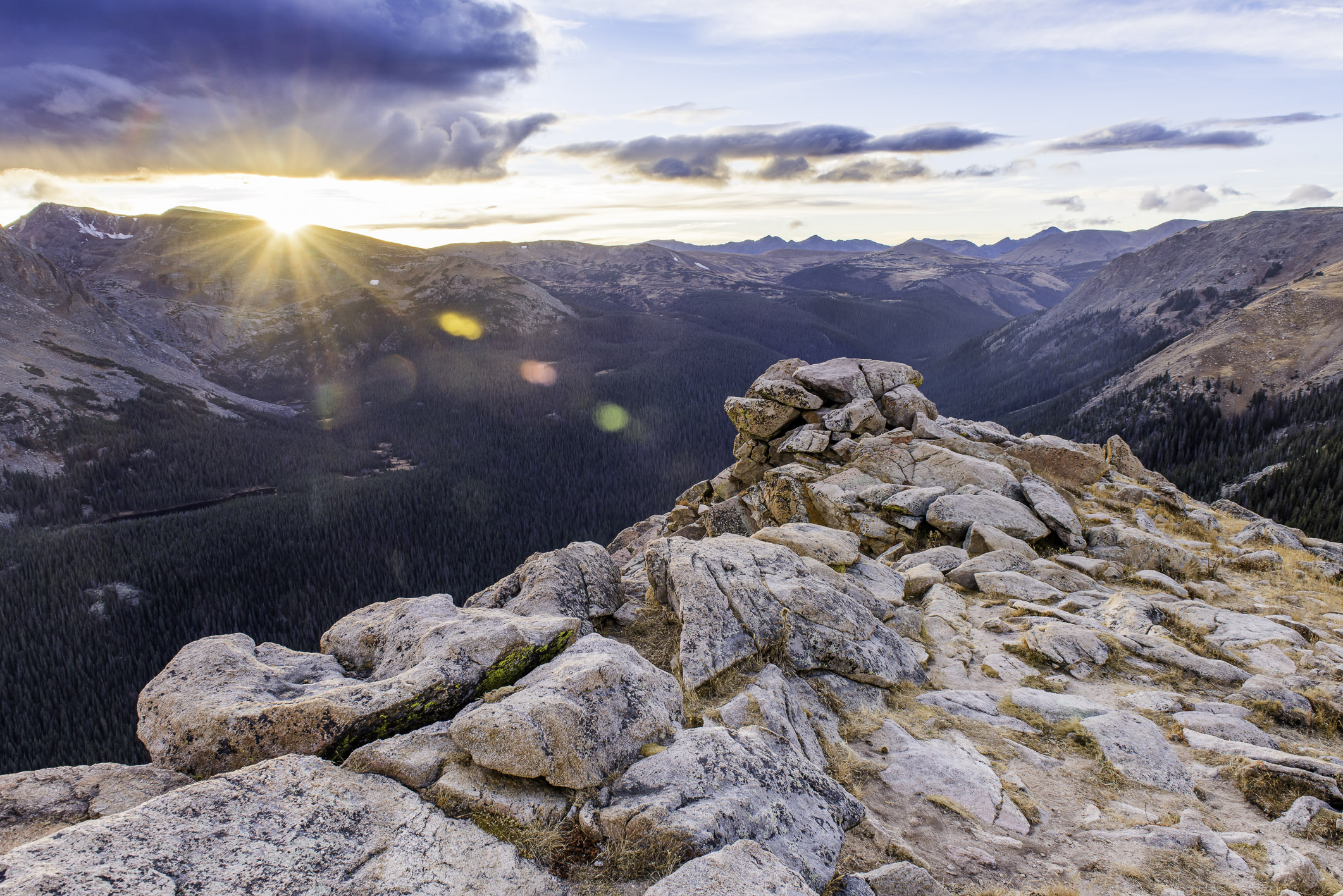The image captures a breathtaking sunrise over a sprawling mountain range, marked by a deep valley blanketed with tall pine trees. At the forefront, tan and brown craggy rocks with black specks and slight grassy foliage extend out over a cliff that plunges sharply into the valley. These rocky outcroppings frame the lower portion of the rectangular photograph, guiding the viewer’s eye towards the central expanse. The valley is steep, and trees begin to populate the mountainsides midway up before thickening at the bottom. Rising majestically in the background, the mountain peaks stretch from the upper left to the upper right, with the tallest peak piercing the emerging sunlight—a bright, warm yellow hue. The sky above is a mix of blue and partially cloudy, with a large dark gray cloud occupying the upper left corner, adding a dramatic contrast to the serene morning light. The overall composition beautifully contrasts rugged cliffs, dense forests, and the soft morning sky, capturing the essence of pristine natural beauty.